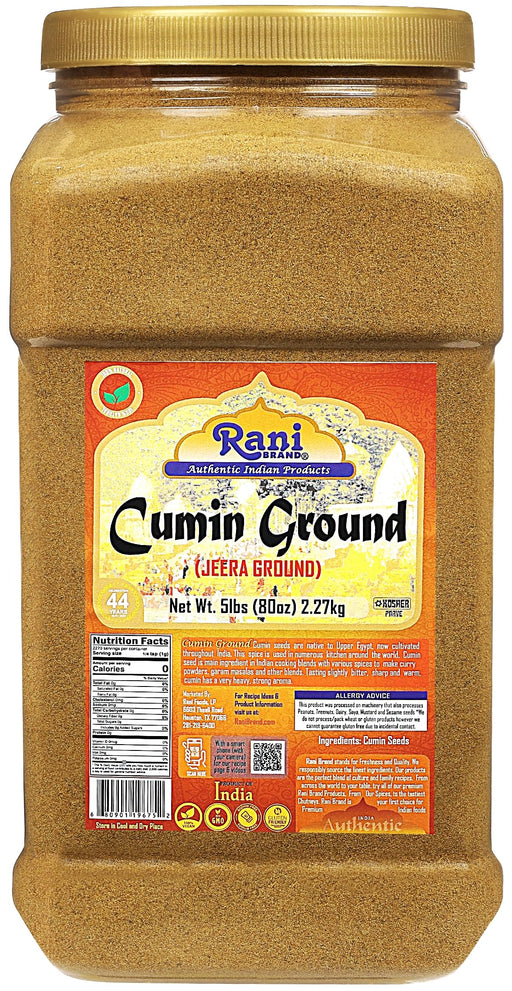This close-up image, set against a white background, features a container of ground cumin from the Rani brand. The jar has a vertically rectangular body, slightly narrower at the base and topped with a rounded, light brown lid. A reddish-orange label, prominently placed on the jar’s front, displays the brand name "Rani" inside a bun-shaped logo, followed by the words "Authentic Indian Products" in a blue bar. Below, it states "Cumin Ground (Jara Ground)" in red, indicating the spice's variant, along with its net weight of 5 lbs (80 oz or 2.27 kg). The left side of the label features nutrition facts, while the right side lists the ingredients and other information in small, hard-to-read white text. At the bottom of the label, the product origin is indicated as "India," with four yellow logos underneath. The jar itself appears to be made of clear plastic or glass.